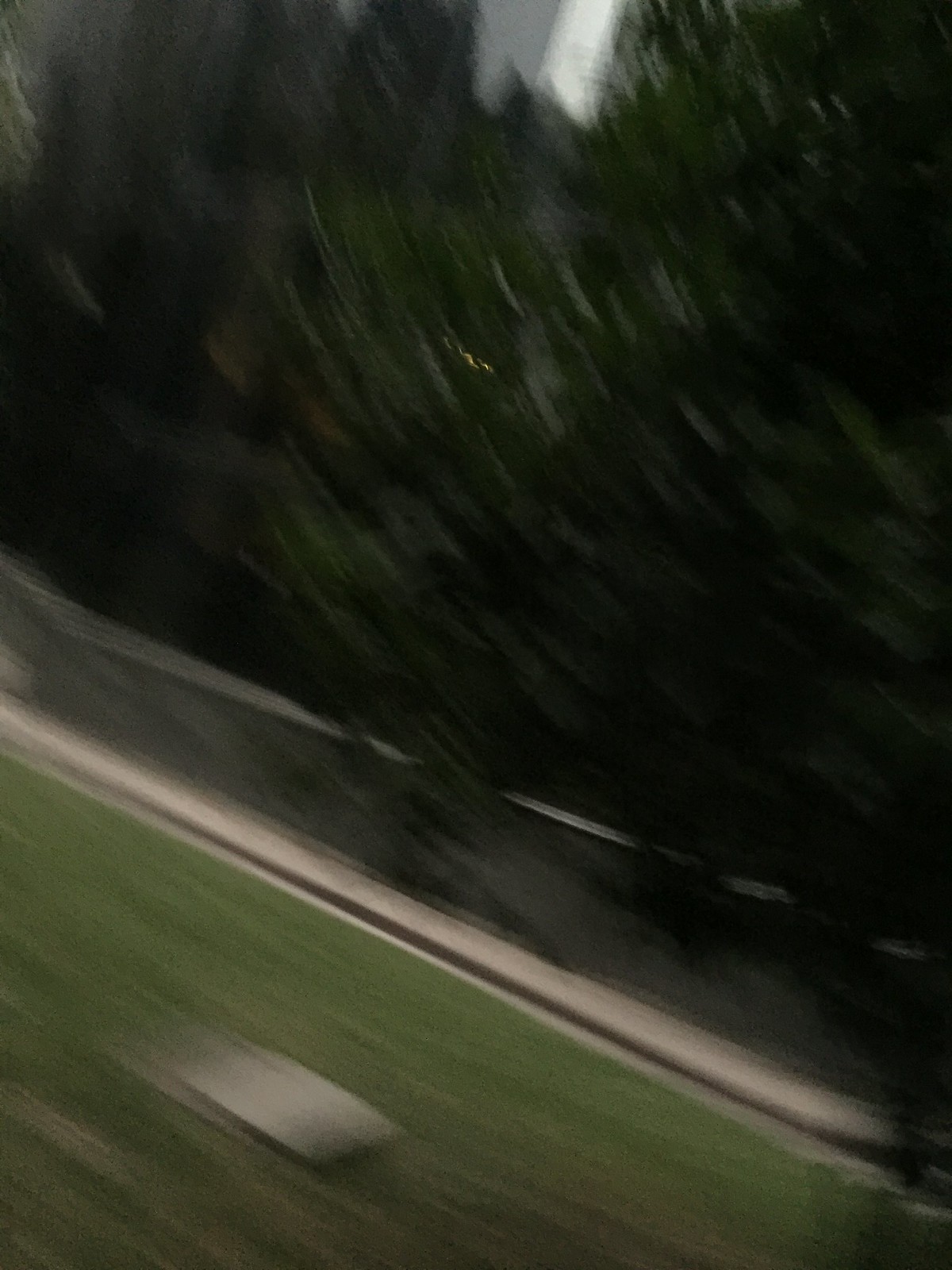In this somewhat blurry action shot, the scene features a lush green landscape with neatly trimmed lawns extending towards the foreground. The vibrant greenery dominates the middle section, complemented by well-maintained hedges and trees. In the very background, towers are faintly visible, adding a structural contrast to the natural setting. The image is marked by distinct white lines running along the edges, enclosing a central black line that runs through the middle. Additionally, a noticeable white square sits prominently near the bottom of the frame, while a gray line subtly divides the green expanse. The image composition suggests a dynamic movement from left to right, with the blend of colors and lines creating a sense of depth and motion.